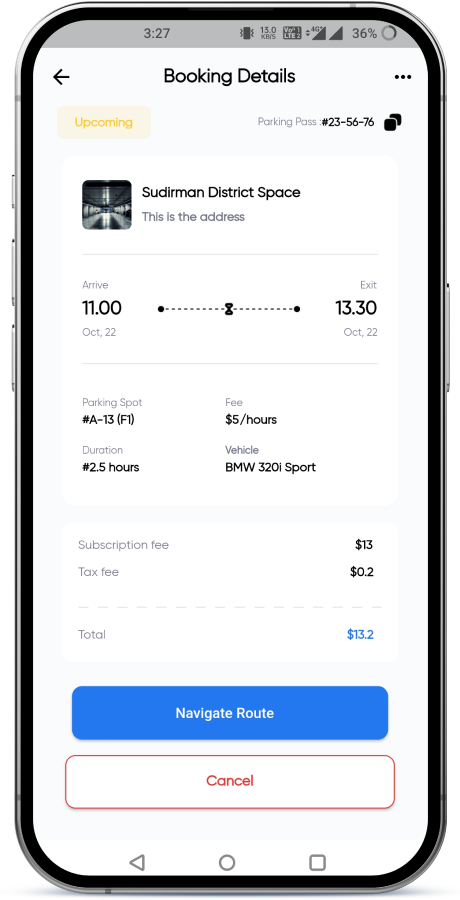The screenshot displayed captures a mobile phone interface, showcasing a booking details page for a parking reservation. The phone's battery is at 36%, and the main focus is the outlined parking reservation. At the top, there is an "Upcoming" section detailing the reservation specifics.

The parking reservation is for "Sued Dreaming District Space," though the exact address is not shown. The booking is for October 22nd, with the arrival time set at 11:00 AM and exiting at 1:30 PM the same day—totaling a duration of 2.5 hours. The parking spot number is specified, and the rate is $5 per hour.

In terms of costs, the parking fee amounts to $12.50 for 2.5 hours, with an additional subscription fee of $13 and a tax fee of $2, bringing the grand total to $27.50. The vehicle listed for this reservation is a BMW 320i Sport.

Below the booking details, there is a prominent blue button labeled "Navigate Route," which provides directions to the parking location. An alternative option to "Cancel" and search for another parking spot is also available.